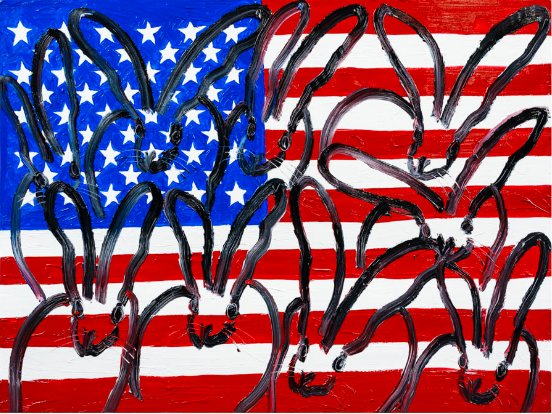The image is a landscape-oriented, hand-painted piece of art prominently featuring the United States flag. The flag, painted on what looks like a white canvas, showcases the iconic blue field with white stars in the upper left corner, and the red and white stripes extending to the right and below. The paint used for the flag is notably thick, with several areas where the red stripes and the blue field are applied in thick, textured globs.

Overlaying this striking flag are approximately eight or nine rabbits, each drawn with a continuous black brush stroke or possibly a black ink pen. These rabbits, positioned from the upper left to the right and along the bottom, are minimalist in design, consisting of simple outlines that reveal round heads, straight-up ears, eyes, noses, and mouth smiles. Unique details such as whiskers appear to be etched into the thick paint, possibly with a tool like a toothpick, adding a unique textural element. The rabbits face the viewer, creating an engaging and whimsical contrast to the patriotic background. The repetitive and neatly aligned rabbits across the flag give the artwork a cohesive yet playful feel.